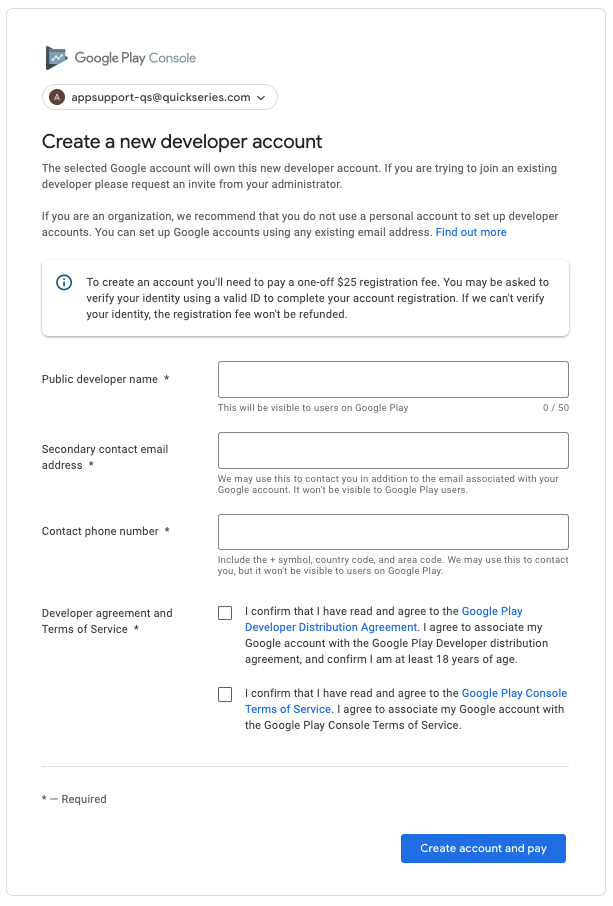The image features a large white box with various elements related to setting up a Google Play Console developer account. In the top left corner, there is a graphical header displaying "Google Play Console." Below this, contained within a long white oval, is the email address "appsupport.qs@quickseries.com" accompanied by a downward-facing arrow.

Directly beneath the oval, bold black text instructs the viewer to "Create a new developer account." Following that, in a lighter black font, it is explained that "The selected Google account will own this new developer account. If you are trying to join an existing developer, please request an invite from your administrator."

A new sentence advises, "If you are an organization, we recommend that you do not use a personal account to set up developer accounts." It adds that you can set up a Google account using any existing email address, followed by a blue hyperlink that says "Find out more."

Below this paragraph is a notification box featuring an exclamation mark inside a circle which states that to create an account, there is a one-off $25 registration fee. It also mentions that you may need to verify your identity using a valid ID and that if identity verification is unsuccessful, the registration fee will not be refunded.

The form fields for account setup are as follows:
- "Public Developer Name" with an empty input box 
- "Secondary Contact Email Address" with an empty input box 
- "Contact Phone Number" with an empty input box 

Additionally, there is a section for agreeing to the "Developer Agreement and Terms of Service" with two checkboxes to confirm agreement with the terms.

An asterisk next to certain fields indicates that those fields are required. Finally, in the bottom right corner, there is a blue button with white text that says "Create Account and Pay."